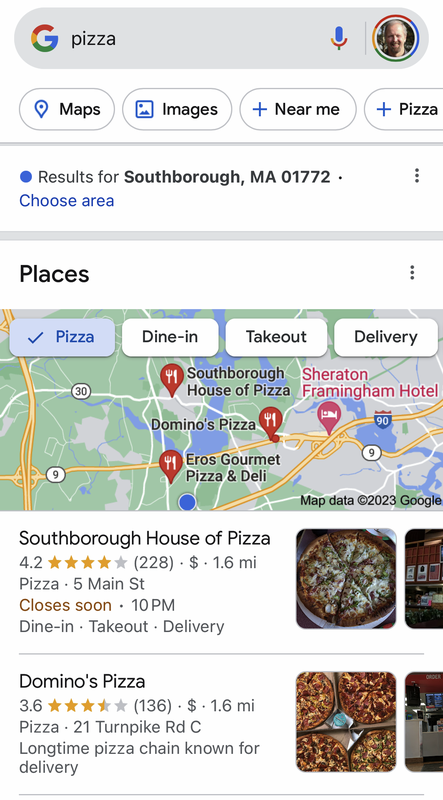This image is a detailed screenshot of a Google search result page with a focus on places to get pizza. The background is off-white with elements organized in a structured layout. 

At the very top of the image, there is a gray oval search bar. On the left side of the bar, a multicolored Google logo (with the characteristic "G") is present. To the right of the logo, in black text, it says "pizza." On the far right of the search bar, there is a multicolored microphone icon and a user profile icon featuring a picture of a middle-aged man with a beard, surrounded by a multicolored edge mirroring the Google logo.

Beneath the search bar are four oval buttons with a white background, each adorned with blue icons on their left side and black text:
1. A pin icon with the word "Maps"
2. An image icon labeled "Images"
3. A blue plus sign next to "Near me"
4. Another blue plus sign beside "Pizza"

Following these buttons, a gray line separates the sections. Below this line, the text reads "Results for Southboro Mass 01772" accompanied by a blue bullet point and the phrase "Choose area" in blue. On the right-hand side of this section are three vertical dots.

Below a wider gray line, the word "Places" is bolded in black in the upper left corner, with another set of three vertical black dots on the upper right. A section of a Google Map is displayed beneath this caption, featuring three rectangular buttons at the top. The first button on the left is blue and says "Pizza" in bolded blue text with a check mark beside it. Next to it, the remaining buttons are white with black lettering, respectively labeled "Dine in," "Take out," and "Delivery."

On the map, there are four red pins, each marked with a white knife and fork icon. The first search result displayed under the map is "Southboro House of Pizza," which has 4.2 stars and is located 1.6 miles away. On the right side of this result are images of a pizza and a dining room. The second search result is "Domino's Pizza," rated at 3.6 stars and also situated 1.6 miles away. To its right are images showing four pizzas in boxes and a counter inside a Domino's outlet.

This detailed breakdown captures the comprehensive view of the Google search results page for pizza places in Southboro, Mass.